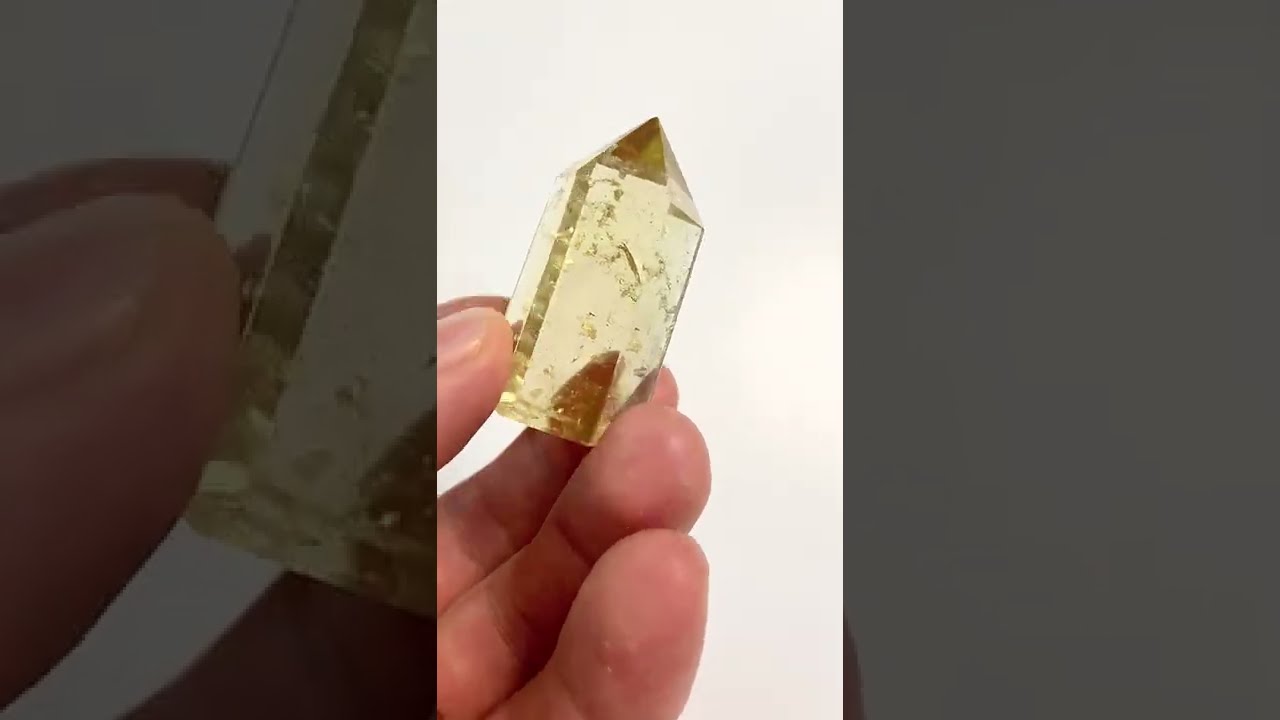In this detailed photograph, a light-skinned individual's hand carefully holds a small, delicate crystal or gem close to the camera. The crystal, which has a translucent, light amber hue with a darker amber tip, is shaped like a tall pyramid with flat sides and a pointed top. The fingers holding the gem are positioned in the lower left-hand corner of the image, offset against a pure white background. The gem appears to have slight imperfections, such as scratches or small air bubbles inside it, adding to its intricate appearance. There is a duplicated section of the image to the left, slightly enlarged and darkened, perhaps intended to show magnification but instead causing some visual confusion. The overall image emphasizes a close-up view of the crystal, highlighting its unique shape and color variations.